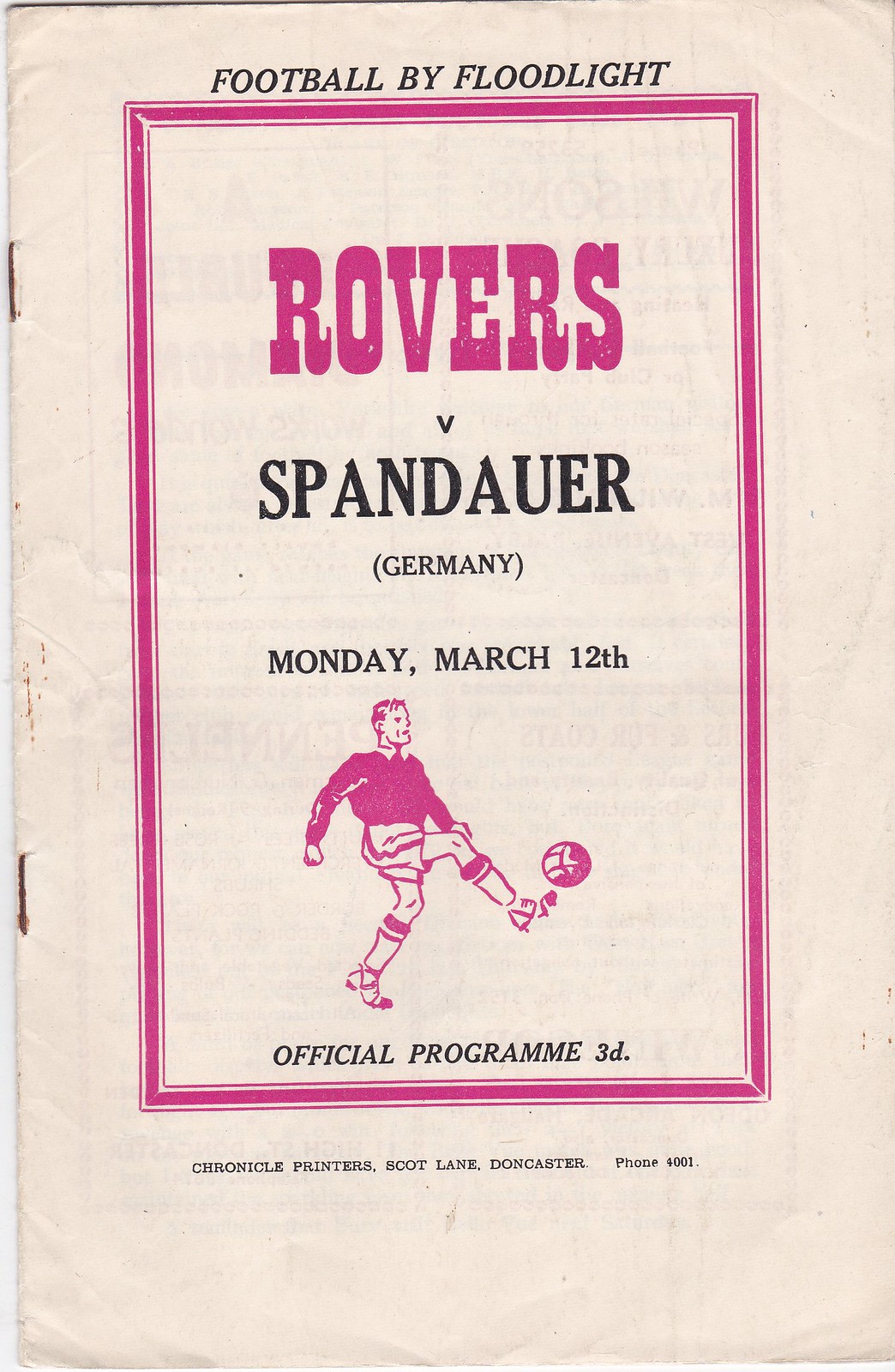The image features the cover of an old football program, primarily on a white background that reveals two rusty brown staples on the left side. Dominating the cover, there is a square section trimmed in pink (sometimes appearing red), with "Football by Floodlight" printed in black text at the top. The headline "ROVERS" is boldly displayed in large pink letters, while "vs. SPANDAUER (Germany)" appears beneath in black text, with "Monday, March 12th" following in the same font. Central to the image is artwork of a football (soccer) player, donned in dark top and light-colored shorts, captured mid-action as he kicks a ball. This figure is rendered in pink, matching the border trim. Below the player, still within the rectangle, the text reads "Official Program 3D" in black. Outside the main highlighted square, the bottom of the program cover includes the text "Chronicle Printers, Scott Lane, Doncaster, phone 4001." Overall, the design includes a harmonious blend of black and pink elements, emphasizing the classic, nostalgic look of a vintage football program.